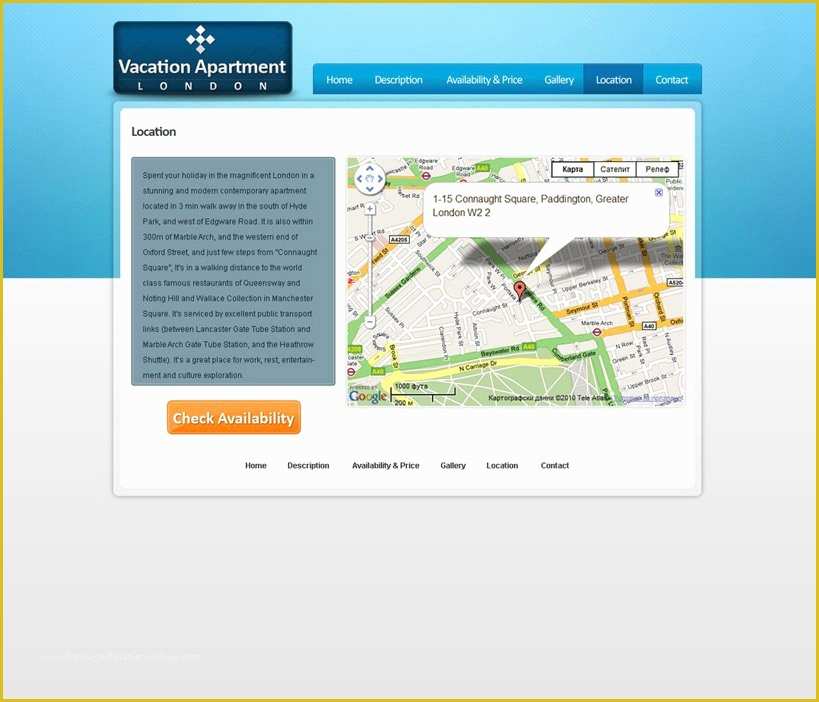**Vacation Apartment in London - A Perfect City Getaway**

**Location:** 1-15 Connaught Square, Paddington, Greater London, W2 2

**Description:** 
Spend your holiday in the heart of London at a stunning and modern contemporary apartment located just a three-minute walk south of Hyde Park and west of Edgware Road. This exquisite apartment is situated within 300 meters of Marble Arch and the western end of Oxford Street, placing you in close proximity to some of London's top attractions.

**Nearby Attractions:**
- **Hyde Park:** Enjoy a leisurely stroll or a picnic in one of the city's most famous parks.
- **Edgware Road:** Discover a variety of shops, cafes, and restaurants.
- **Oxford Street:** Shop till you drop in one of the world's most famous shopping destinations.
- **Queensway and Notting Hill:** Explore world-class restaurants and vibrant nightlife.
- **Wallace Collection:** Visit the remarkable art collection in Manchester Square.

**Transport Links:**
- **Tube Stations:** Conveniently serviced by Lancaster Gate and Marble Arch Tube stations.
- **Heathrow Shuttle:** Easy access to Heathrow Airport.

**Features:**
This apartment is ideal for travelers looking to balance work, rest, entertainment, and cultural exploration. With its modern amenities and prime location, it offers a perfect base for experiencing all that London has to offer.

**Availability:** [Check Availability]

Explore this premium vacation apartment and plan your ideal London getaway today!